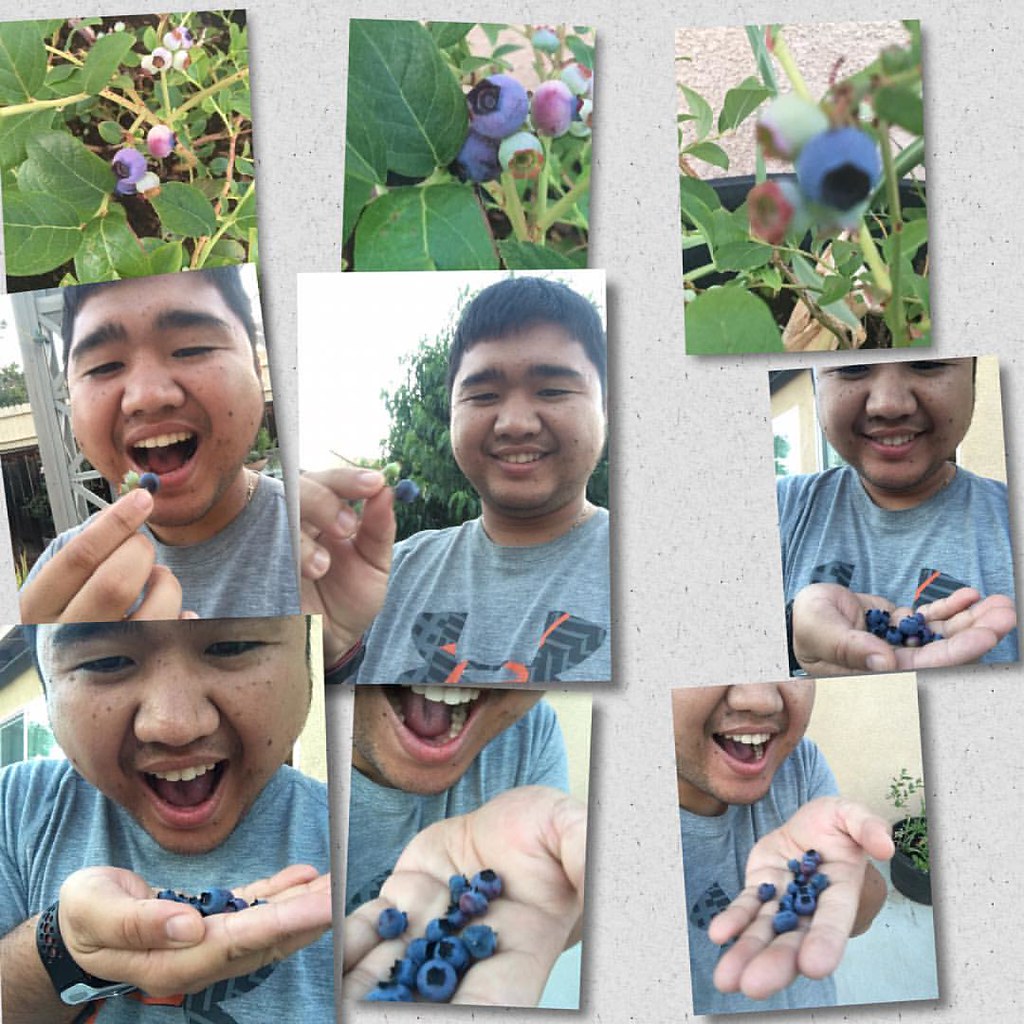The image is a collage of nine interconnected photos featuring a sequence of blueberry-eating moments. The top row comprises three progressively closer close-ups of a blueberry plant, showcasing a mix of ripe blue and unripe green berries amidst lush green leaves. The middle row introduces an Asian man with a chubby face and short hair wearing a gray Under Armour t-shirt. In the first middle-row photo, he faces the camera with a smile, holding a blueberry close to his mouth. The next photo in that row shows him holding a blueberry towards the camera, still smiling. The final middle-row photo captures him with his head slightly cropped, proudly displaying a palm full of ripe blueberries. In the bottom row, he leans forward, appearing ready to devour the handful of blueberries, his mouth wide open in anticipation. The following photos repeat this action from slightly different angles, with a potted plant occasionally visible in the background.